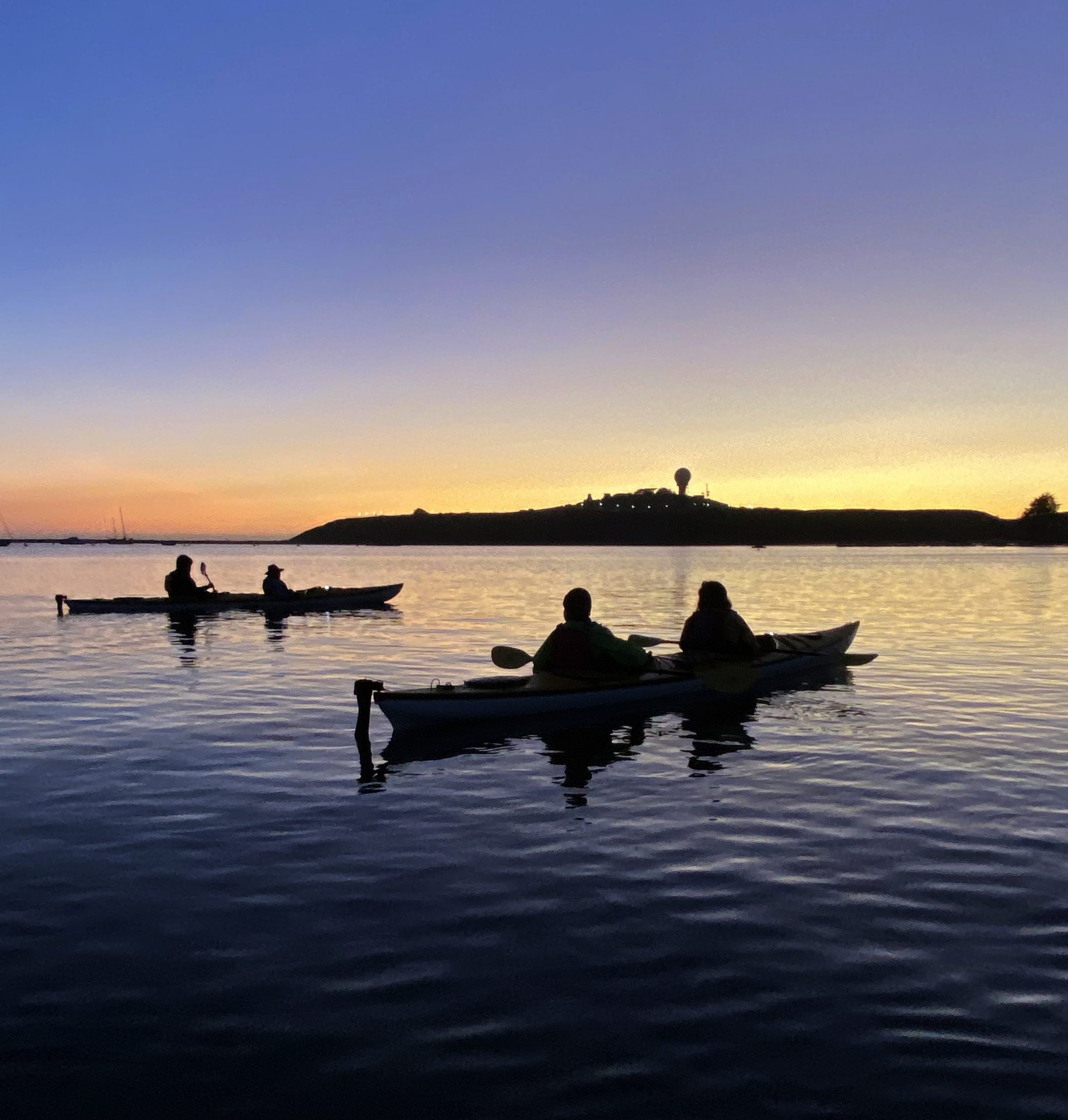In the image, we see a tranquil ocean scene during dusk, characterized by a mesmerizing gradient sky that transitions from a rich, light indigo at the top to vibrant yellows and oranges near the horizon as the sun sets. The navy blue and slightly rippled water reflects these stunning colors, creating a peaceful atmosphere. In the foreground, two canoes glide smoothly across the calm water. Each canoe holds two people, all silhouetted against the sunset's golden reflection, making their individual features indiscernible. They are paddling gently, though there appear to be small outboard motors attached to the back of each canoe. In the background, a mountain rises, adding a majestic touch to the landscape. Additionally, there's a prominent hill along the horizon, featuring a water tower and a building at its center, further enriching the scene's detailed beauty.